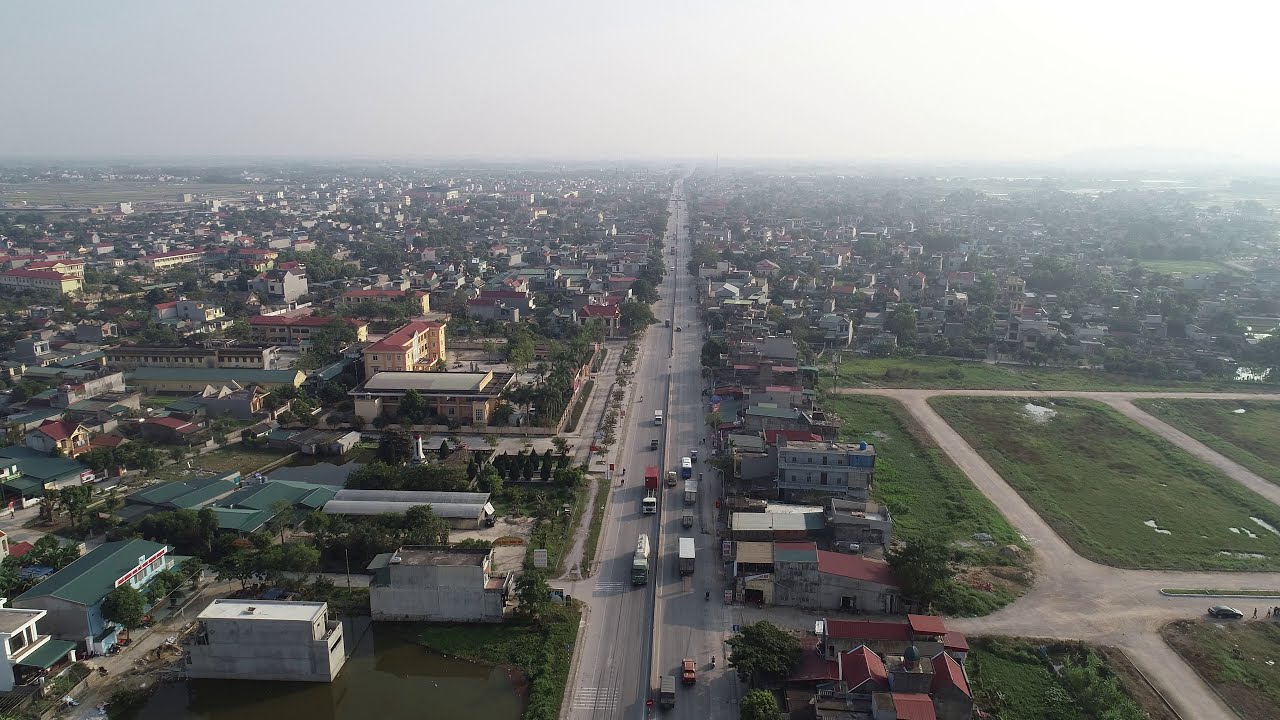This is a full-color aerial photograph taken outdoors on a sunny, yet possibly foggy day. The image showcases a town rather than a city, as seen from above. Dominating the central part of the image is a four-lane road running vertically from the bottom towards the top. Several vehicles can be observed traveling along this road.

Flanking the central road are a variety of buildings, with a larger concentration of structures on the left side. These buildings vary in height but do not surpass three or four stories. Among them, there appears to be a hotel. The roofs of the buildings are diverse, displaying hues of red, green, and flat grey.

On the right-hand side of the image, there are fewer buildings interspersed with open fields and roads outlining rectangular parcels of grass. The overall palette of the image includes an array of colors such as red, green, gray, brown, white, yellow, and orange, with different shades of green and blue contributing to the scene’s vividness.

The photograph captures a blend of residential and commercial areas, providing a detailed and vibrant overview of the town set against the backdrop of a clear, bright day. There is no text visible within the image.